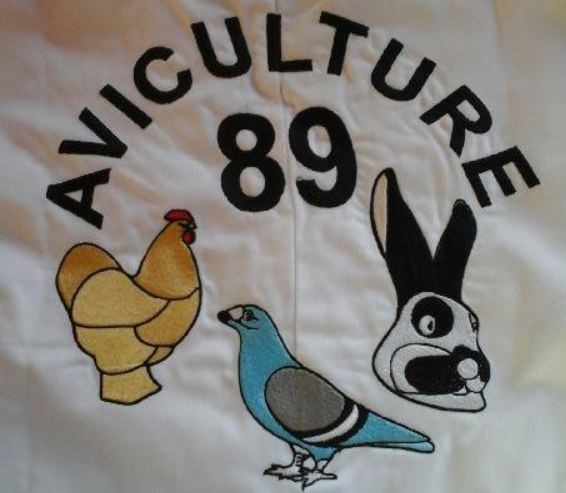The image is a detailed close-up of a white fabric, possibly a piece of clothing or a blanket, with a centered design. The design features black arched text at the top that reads "Aviculture" and a large black number "89" beneath it. Below the number are three animal illustrations: a chicken on the left, a blue bird in the middle, and a rabbit's head on the right. The fabric appears to be soft, and the image captures vivid colors, including black, white, orange, yellow, red, and light blue. The layout suggests a deliberate design possibly used in clothing, and the high level of zoom implies it might be an advertised item for online display or on a shelf.